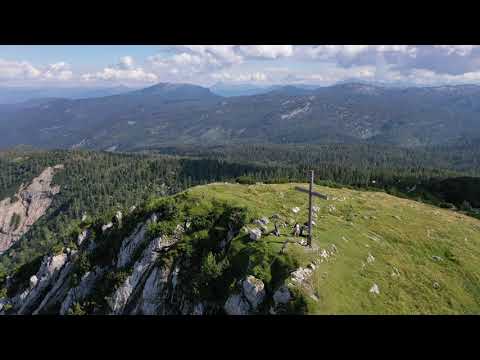An aerial photograph showcases a stunning nature area dominated by a large wooden cross mounted atop a verdant hill or mountain peak. The image, though grainy, captures the essence of the rugged landscape, characterized by green foliage interspersed with rocky slopes. Blue skies punctuated with clouds hang over multiple mountain peaks in the distance. The photograph appears to have been taken from a drone or aircraft, offering a panoramic view of the serene, untouched wilderness with no signs of civilization except for the prominent cross. There are indistinct shapes near the cross, possibly people, adding a subtle human element to this wilderness scene glowing under the bright sunshine.